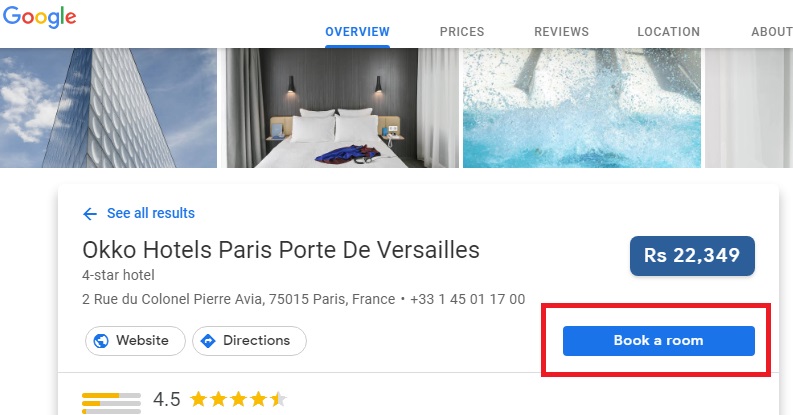The image showcases a Google search results page for "Poco Hotels Paris Porte de Versailles." At the top of the page, there are several tabs labeled "Overview," "Prices," "Reviews," "Location," and "About." The "Overview" tab is currently selected. Below these tabs, a series of thumbnail images are displayed, including a swimming pool, a hotel room, and the hotel building itself. Beneath these images, there is a link that says "See all results." The main text on the page reads "Poco Hotels Paris Porte de Versailles," indicating it is a four-star hotel. Below this, the hotel's French address is provided.